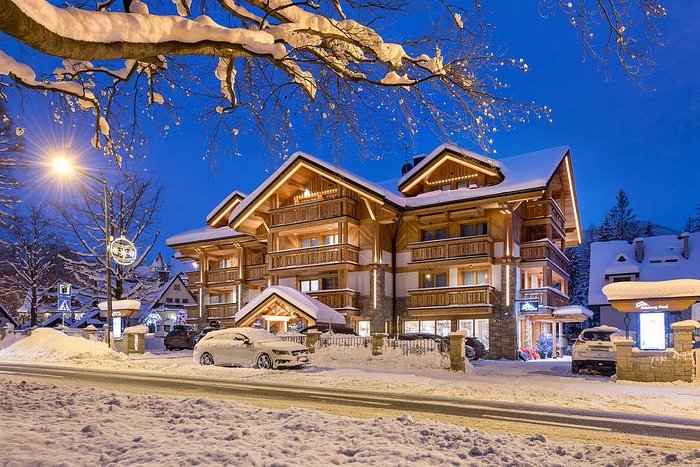This photograph captures a picturesque log cabin-style hotel or B&B, set in a snow-covered ski village, possibly in Colorado. The three-story wooden structure features multiple balconies with wooden railings, and its triangular roofs and log construction give it a rustic, mountain lodge appearance. The building is flanked by a neighboring establishment with a neon sign, indicating it is open to the public. The scene is enveloped in heavy snowfall, blanketing the ground, roofs, and nearby trees. A strip of road and several cars, heavily covered in snow, are visible in front of the building. The setting is during twilight, with a deep blue sky providing a backdrop, and some lights are already illuminated, hinting at the approaching night.